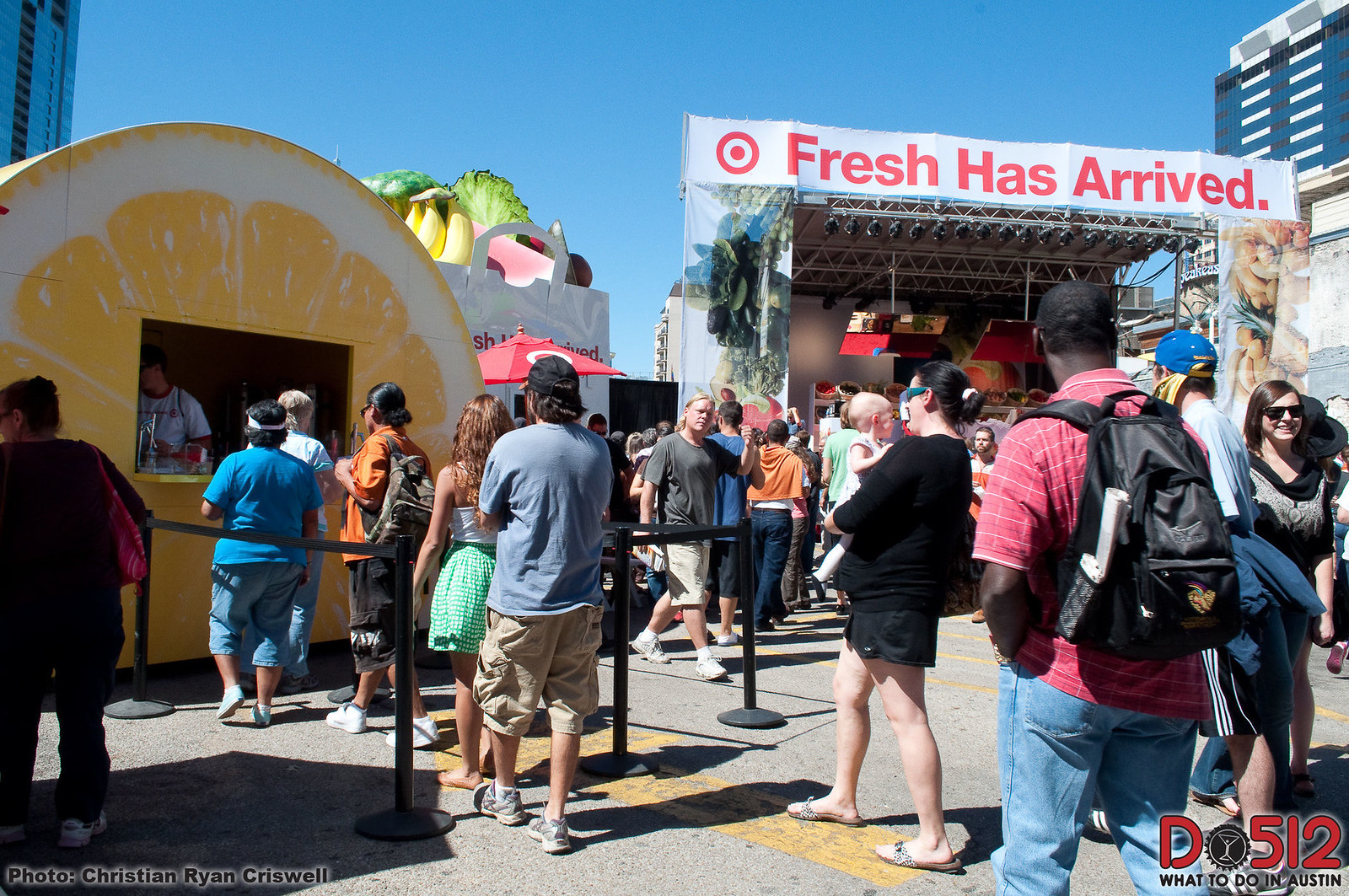The image captures a bustling scene at an event where a large group of people is gathered. In the foreground, a line of individuals, most sporting backpacks and baseball hats, is queued up at a refreshment stand. The stand is whimsically decorated to resemble a large slice of citrus, with a white border and a bright yellow center, indicating it's possibly a lemonade stand. Inside the stand, a person is attending to the customers. Particularly notable is a woman right in front of the viewer holding a small baby.

In the background, a towering, elaborate display mimics an oversized shopping bag filled with an array of fruits and vegetables such as bananas, broccoli, and lettuce, as well as a watermelon slice peeking out. This display is about a story and a half tall, serving as an eye-catching advertisement.

To the right of the scene stands a stage adorned with numerous stage lights and colorful graphics of fruits, vegetables, or possibly flowers flanking it. Prominent on the stage is the Target logo along with a sign bearing the slogan "Fresh Has Arrived". Underneath the archway of the stage, there appear to be baskets artfully tilted to showcase a bountiful array of produce, adding to the event's theme of freshness and health.